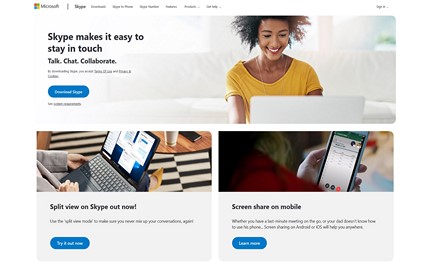The image depicts a Microsoft webpage, with the familiar Microsoft logo comprising four squares in green, blue, red, and yellow located at the top left corner. Tabs are visible at the top but are unreadable. In the top right corner, there is a "Sign In" button. The page has a white background.

On the left side, there is a black text that reads: "Skype makes it easy to stay in touch – talk, chat, collaborate." Below this text is a prominent blue button with white text that says "Download Skype."

To the right of this text, there is an image of a woman wearing a necklace and a yellow T-shirt, intently staring at a white laptop. She is seated on a white couch.

In the bottom left section of the webpage, there is an image of another female looking at a black laptop displaying the text: "Split View on Skype – Out Now. Try it Now." Beneath this, there is a blue button.

In the bottom right section, there is an image of a person holding a phone with the Skype application open. The phone's screen shows various buttons related to Skype. Below this image, there is a description that states: "Screen Share on Mobile. Learn More." The "Learn More" button is also blue.